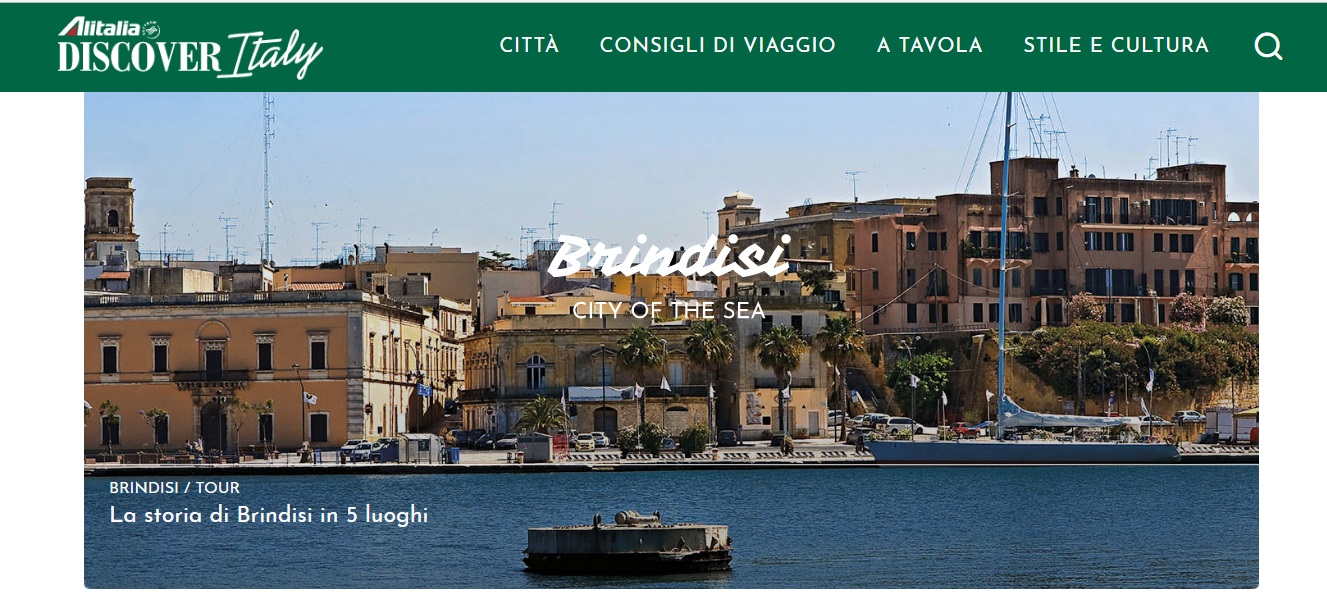This image is a horizontally aligned rectangle, designed as an advertisement for Italy, likely a screenshot of a tourism website. At the top, a green bar spans the width of the page, featuring a brand insignia on the left that reads "Alitalia," followed by the slogan "Discover Italy" in white letters. Adjacent to this, to the right, are navigation options in Italian: "Città," "Consigli di Viaggio," "A Tavola," and "Stile e Cultura," culminating in a small search icon represented by a magnifying glass on the far right.

Beneath this header is a picturesque photo depicting a charming Italian scene. The background showcases an array of buildings, including two-story apartment structures with rectangular windows on both floors, a central cluster of traditional stone buildings, and a taller condominium complex. Palm trees dot the landscape. 

The tranquil blue water in the foreground, rippling gently, suggests the photograph was taken from a boat. A large sailboat with a tall mast is anchored by the shore. Overlaying the scene in white font are the words "Brindisi" and "City of the Sea," with additional text in the lower left corner that reads "Brindisi/Tour," and "La Storia di Brindisi in cinque Luoghi," enhancing the inviting portrayal of the historic seaside town.